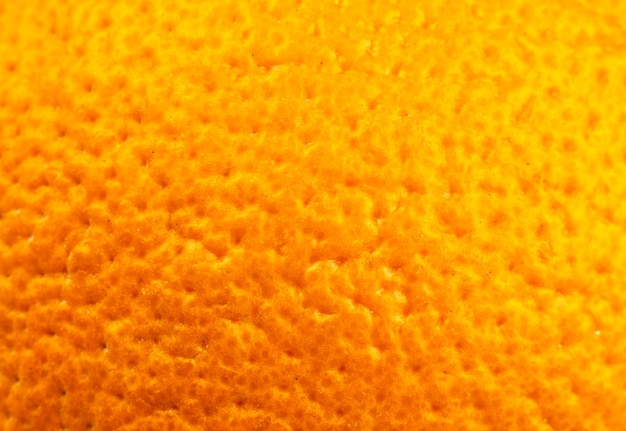This photographic image presents a horizontally aligned rectangular close-up of the textured skin of an orange, filling the entire frame without any border or text. The surface displays a gradient of colors, starting with a deep, bright orange in the bottom left-hand corner that transitions to a lighter yellowish-orange towards the upper parts of the image, with the top left-hand corner appearing almost yellow. The peel's texture is dotted with uniformly sized, small pockmarks or dimples, contributing to its slightly bumpy appearance. The most defined details are visible in the bottom left corner, while some areas of the image appear slightly out of focus, enhancing the sense of depth and realism in this highly detailed and vivid depiction of the orange peel’s surface.